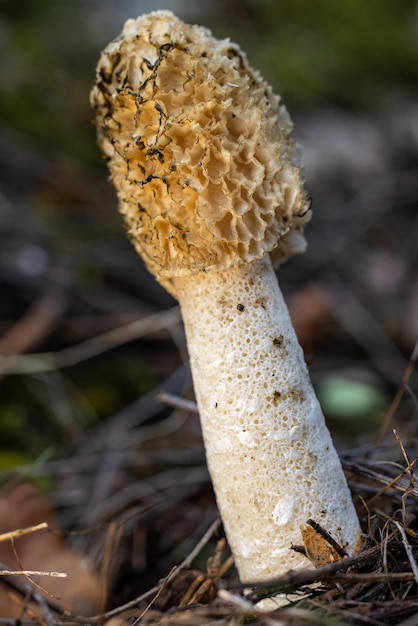This close-up photograph captures a morel mushroom growing out of the ground. The mushroom features a thick, ivory-colored stem with a spongy texture, punctuated by tiny holes, resembling a sponge. The cap of the mushroom is distinctly vertical, more narrow and tall, with an ovular shape. It has a unique wavy texture with a golden brown to orange-ish yellow hue. There's a subtle flaky and slightly burnt appearance at the tips, suggestive of brownish outlines. The high-quality image reveals the mushroom in sharp focus against a blurred background, enhancing its intricate details. Surrounding the morel are various sticks, dark brown twigs, and some ground debris, but no visible insects. The vibrant photo, taken in daylight, immerses the viewer in a natural forest floor setting.